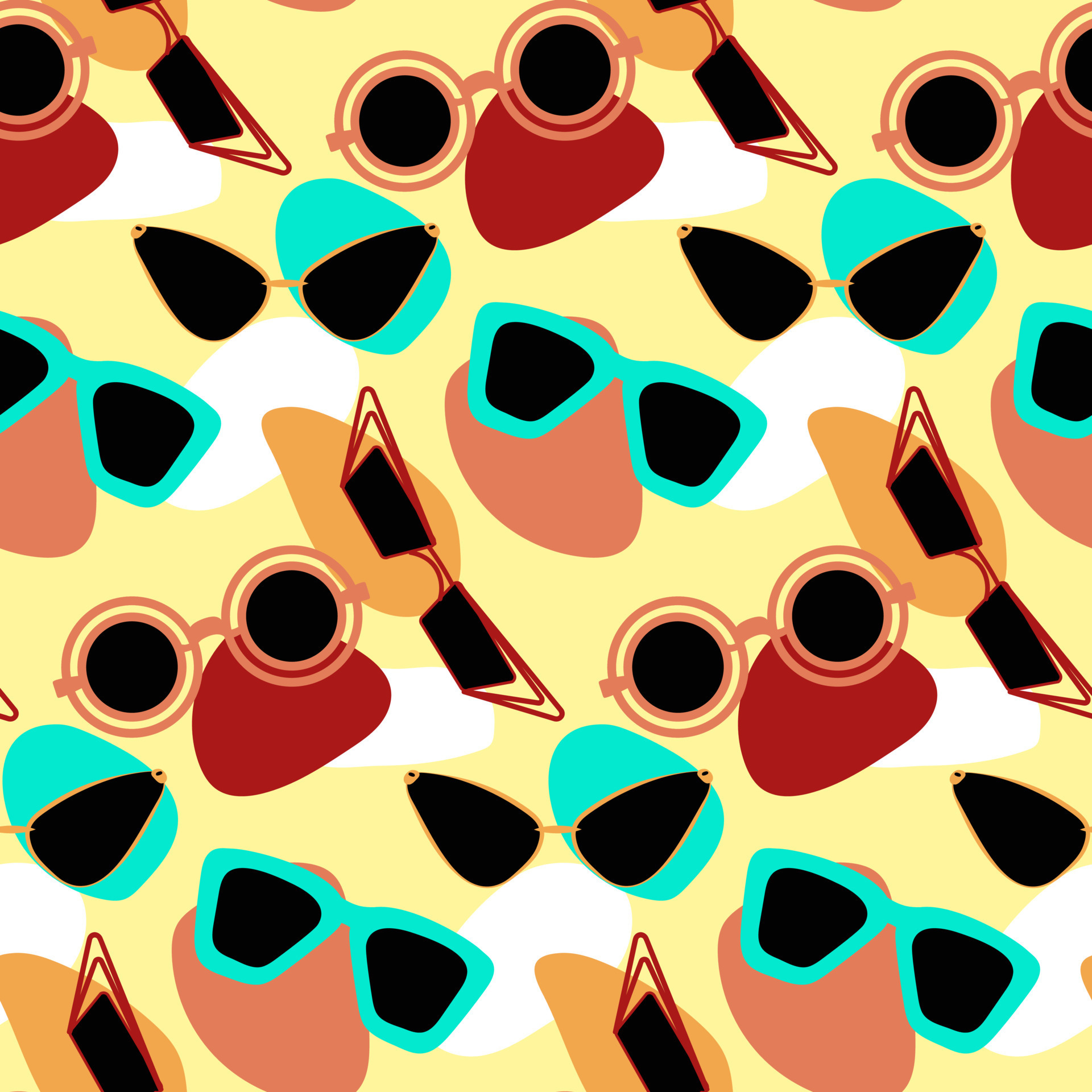The image showcases an artist's rendition of various sunglasses set against a textured, yellowish-beige background adorned with splotches of white, red, and blue. The vertically rectangular artwork features no borders or text, focusing solely on the eclectic assortment of eyewear. Sunglasses of different shapes and sizes are scattered somewhat evenly across the piece, creating a rough, visually appealing pattern. Among the assortment, one can spot round frames with concentric orange circles enclosing black lenses, turquoise blue frames, rectangular red frames with triangular edges, and delicate yellow-orange frames. The dominant color palette includes black lenses paired with frames in red, blue, yellow, and occasionally gold, all contributing to a vibrant, multi-color visual experience.